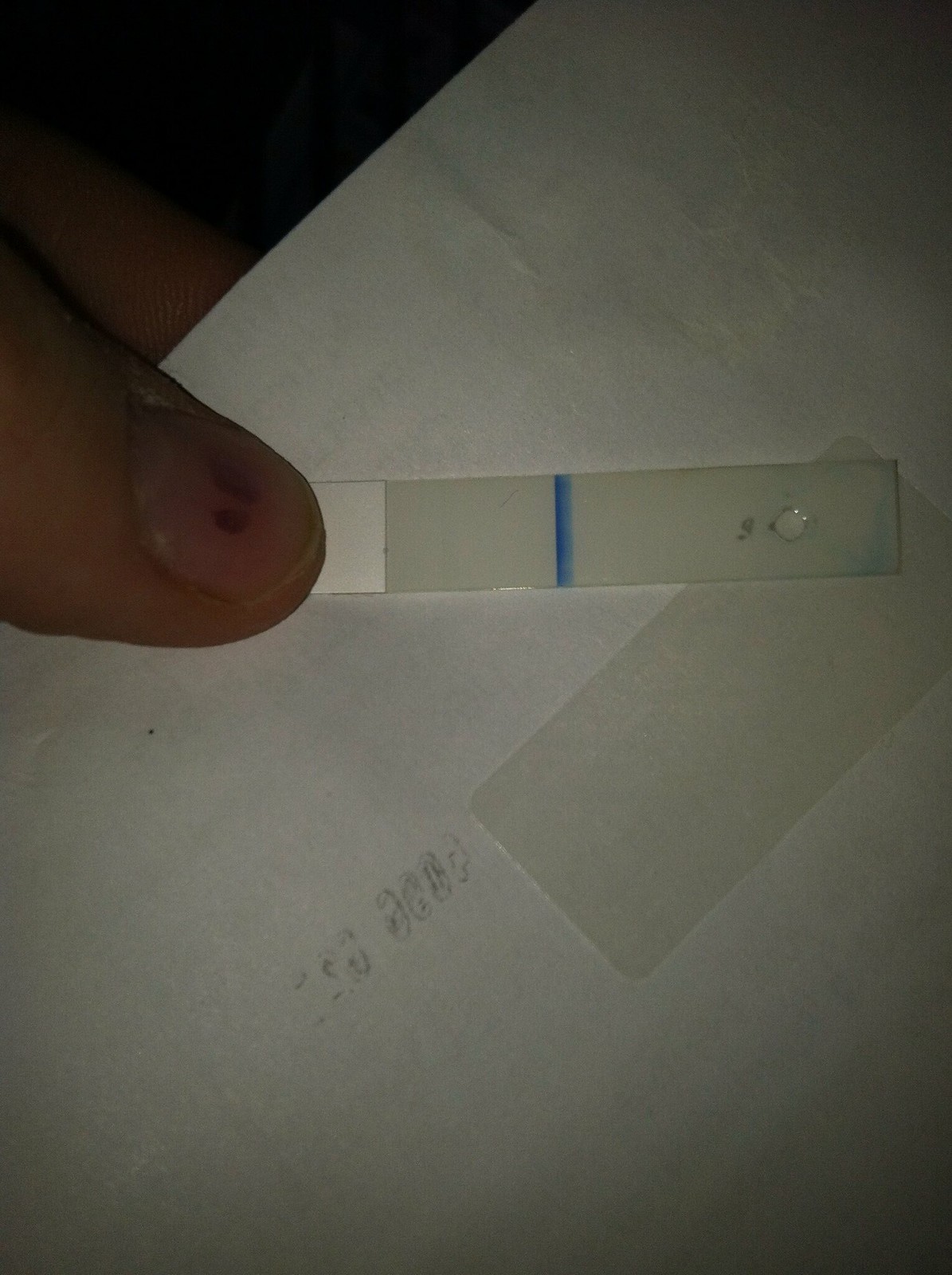In this image, a person is holding a white piece of paper which occupies most of the frame. Their left hand, identifiable by either their thumb or pointer finger, is seen in the top left corner pressing down on the paper. The thumbnail appears unclean, with noticeable black, brown, or red marks. The paper they're holding shows faint, indistinguishable text bleeding through from the other side, possibly representing numbers or characters from another language.

Centrally placed on the paper is a plastic-like object, resembling a sticker, with another overlapping rectangular sticker towards the side. This rectangular sticker features a small circle on its right side, and a horizontal blue line is visible within the rectangle. A white element, difficult to distinguish but reminiscent of a clock hand or a movable part, is positioned beneath the person's thumb. The overall composition is dominated by various shades of white, making some details challenging to discern.